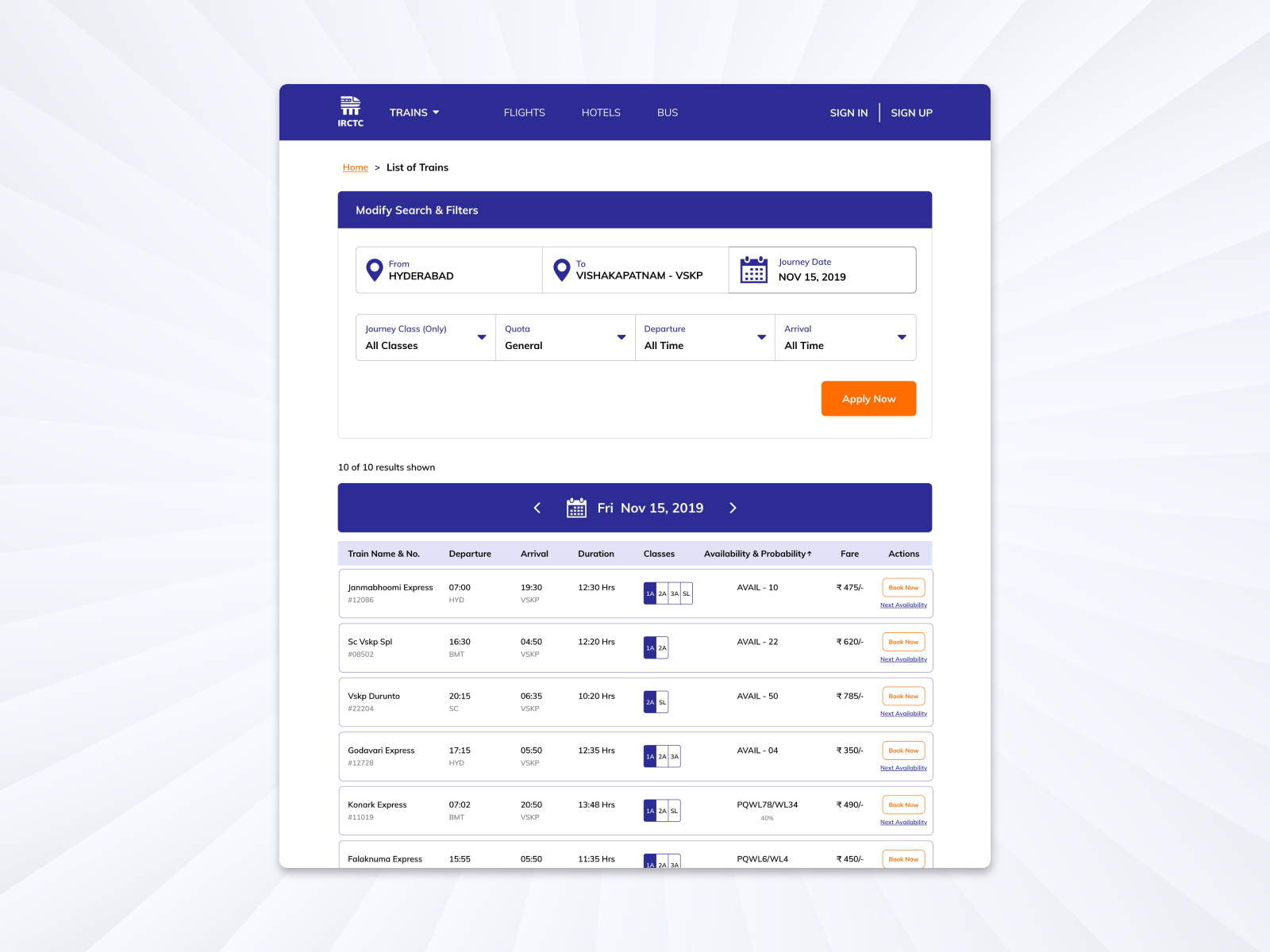The image appears to be a screenshot of a train booking page from the IRCTC (Indian Railway Catering and Tourism Corporation) website. The top section is adorned with a blue background featuring the IRCTC logo marked with a small train emoji. Adjacent to the logo, the menu options listed in white text are "Trains," "Flights," "Hotels," "Bus," and "Sign In/Sign Up."

Beneath this header, the interface transitions to a white background. The navigation bar includes the options "Home" in red and "List of Trains" in black. The title bar is blue, containing white text options "Modify," "Search," and "Filters."

The search parameters for the journey are demarcated clearly with icons. Two location emojis designate the route: "From Hyderabad" to "Vishakhapatnam (VSKP)." A calendar emoji indicates the journey date, which is November 15, 2019. Further options fall under dropdown selections for various criteria including "Journey Class" with an option for "All Classes," "Quota" set to "General," and both "Departure" and "Arrival" times set to "All Time."

An orange box with white lettering on the bottom right prompts users to "Apply Now." Below this, the text indicates "10 out of 10 results shown" for Friday, November 15, 2019. The detailed results section, though partially truncated in the image, displays columns with headers for "Train Name and Number," "Departure," "Arrival," "Duration," "Classes," "Availability and Probability," "Fare," and "Actions." Out of the ten results, only six train entries are visible in the screenshot. The specifics of these entries are not fully legible due to small font size.

Overall, the image captures the structured and user-friendly layout of the IRCTC train booking interface, designed to facilitate easy booking and travel planning for users.